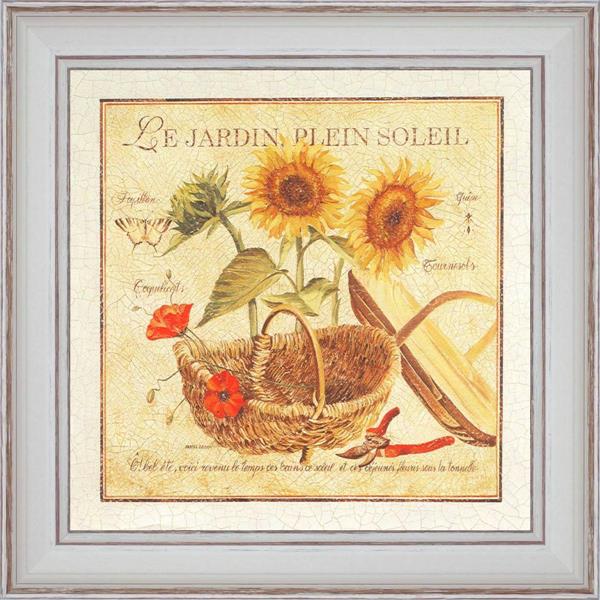The image depicts a framed painting with a white-gray wooden frame and a cream-colored mat, giving it a nearly square appearance despite being a bit more vertical. Inside the frame, the painting features a darker cream background with a detailed composition. Central to the artwork is a woven brown basket, which contains a few red flowers and a pair of silver flower clippers with red handles lying at its base. Behind the basket stand two prominent sunflowers with orangey-yellow petals encircling their reddish-orange centers, accompanied by green stems and leaves. A green sunflower bud is also visible on the left side of the composition. Above the scene is the text "Les Jardins, PLEIN SOLEIL," while additional cursive text runs across the bottom, although it is too small to be legible. A small butterfly is subtly included in the details of the painting.